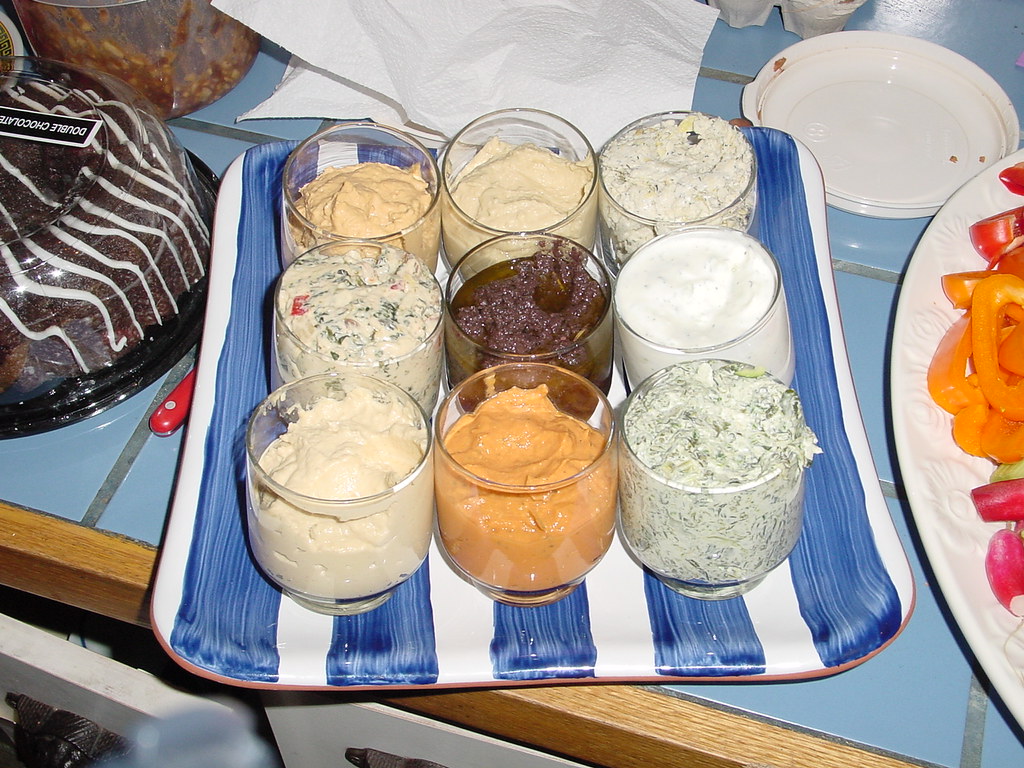This image showcases a vibrant party setup on a blue tiled countertop with a light-colored wood border. At the foreground, there is a striking blue and white hand-painted ceramic tray featuring nine uniformly sized, low-slung cocktail glasses filled with a variety of dips and sauces. The dips range in color, including shades of medium brown, light brown, greyish green, dark browny yellow, pure white, light cream, mustard terracotta, and green-grey, suggesting varieties like spinach dip, anchovy dip, sour cream, queso, and aioli mayo.

To the left of this central display is a dark chocolate bundt cake with white drizzle, labeled "double chocolate." On the right, a white ceramic dish, adorned with an embossed floral pattern, holds an array of sliced vegetables including golden bell peppers, radishes, and celery. Scattered around the table are napkins and paper towels, adding to the casual, festive atmosphere. The table itself is framed by white drawers emerging from its front edge.